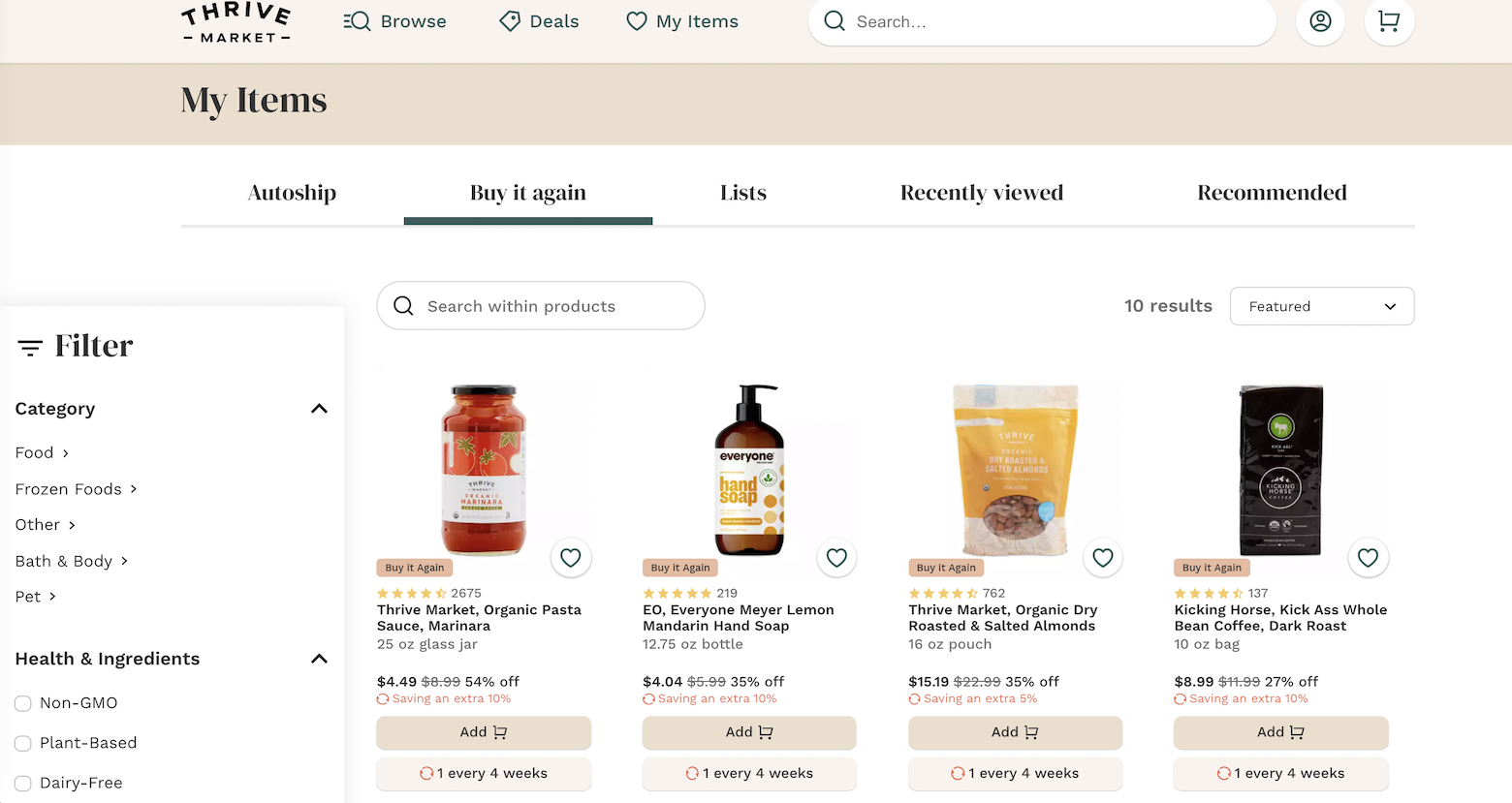A screenshot from the e-commerce website, Thrive Market, showcases its user interface in detail. At the top, a white navigation menu lists options: "Browse," "Deals," and "My Items," accompanied by icons of a magnifying glass, a price tag, and a heart, respectively. Adjacent to these is a search field, a profile icon, and a shopping cart icon.

Beneath this, there's a horizontal navigation bar with "My Items" highlighted in bold. Below these options are additional tabs: "Auto-Ship," "Buy It Again," "Lists," "Recently Viewed," and "Recommended," with "Selected For You" underlined.

A vertical filter menu on the left side categorizes items under headings like "Category" with subcategories such as "Food," "Frozen Foods," "Baby Food," and "Pets." Another bold menu under "Health and Ingredients" lists filter options like "Non-GMO," "Plant-Based," and "Dairy-Free."

The main content area to the right displays ten product results, though only four are visible in the screenshot. Each product listing features an image of the item, a "Buy It Again" button, the product name, price, star rating, and an "Add to Cart" button. Visible products include: 
- Organic pasta priced at $4.99,
- Lemon mandarin hand soap in a brown pump bottle,
- A packet of organic dry roasted salted almonds,
- Kicking Horse Kick-Ass Whole Bean Coffee in a black bag.

The star ratings are partially obscured, rendering them unreadable.